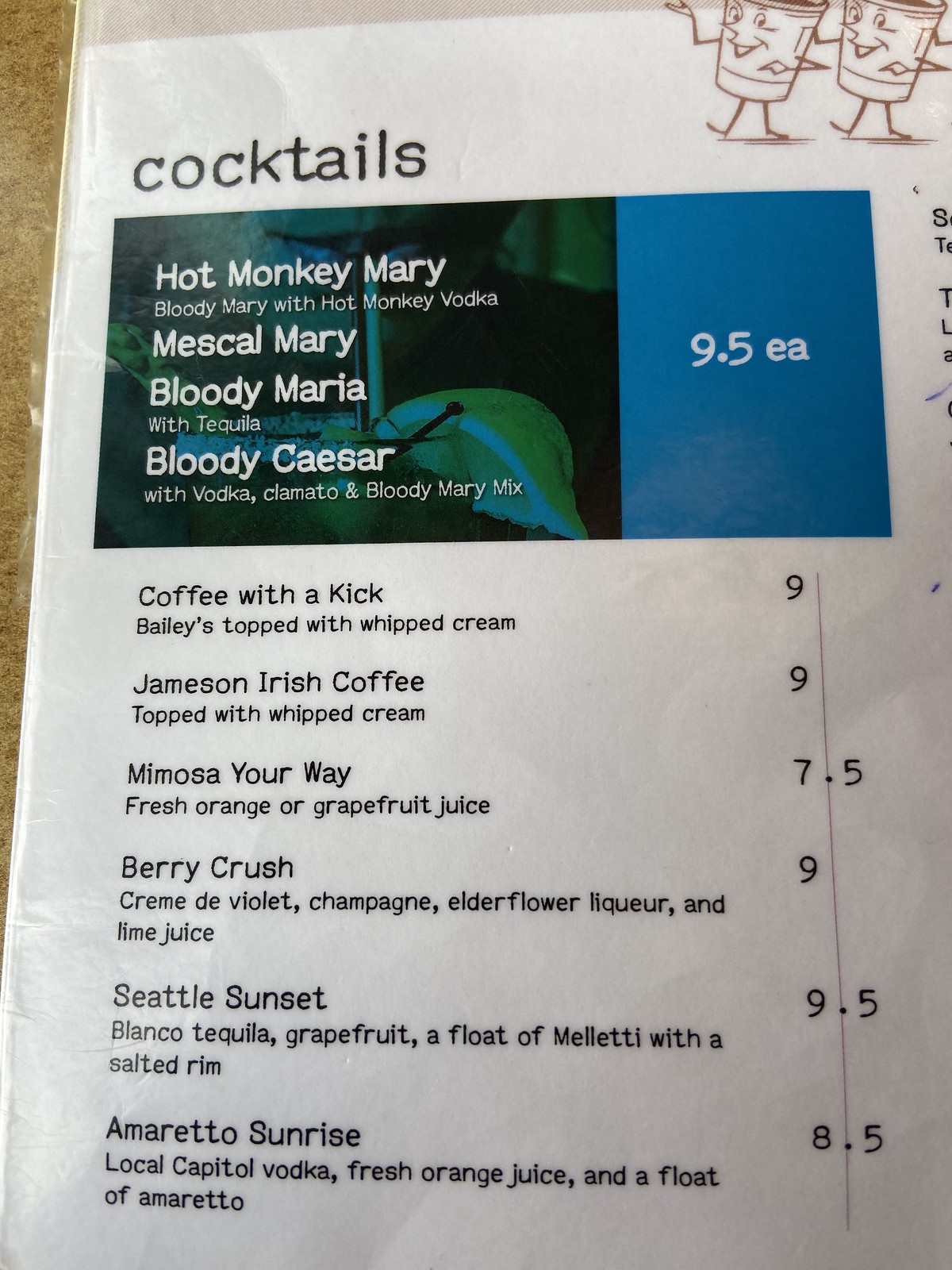The image depicts a laminated drink menu, specifically showcasing the cocktail selections on a white paper background. The visible portion of the menu appears to be the top left section, leaving out the other half or three-quarters of the full menu. 

In the top right corner, there are two animated coffee cups, drawn in brown ink, that appear to be dancing and smiling, adding a playful element to the menu.

At the top left, the word "Cocktails" is prominently printed in black typeface. Just below this headline, there is a colorful box containing a dark background on the left side, featuring a lemon wedge and a list of cocktail names in white font:

1. **Hot Monkey Mary** - A Bloody Mary with Hot Monkey Vodka.
2. **Mescal Mary**
3. **Bloody Maria** - Made with Tequila.
4. **Bloody Caesar** - Contains Vodka, Clamato, and Bloody Mary Mix.

Attached to this box on the right side is a blue section with white text that indicates each of these cocktails is priced at $9.50.

Below this colorful section, on the plain white background, another set of drink options is listed in black typeface under the heading "Coffee with a Kick":

1. **Bailey's topped with whipped cream** - Priced at $9.00.
2. **Jameson Irish Coffee** - Also topped with whipped cream, priced at $9.00.
3. **Mimosa Your Way** - Fresh orange or grapefruit juice, priced at $7.50.
4. **Berry Crushed** - Contains Crème de Violette, Champagne, Elderflower Liqueur, and Lime Juice, priced at $9.00.
5. **Seattle Sunset** - Made with Blanco Tequila, Grapefruit, and a Float of Mileti with a Salted Rim, priced at $9.50.
6. **Amaretto Sunrise** - Local Capital Vodka, Fresh Orange Juice, and a Float of Amaretto, priced at $8.50.

Please note, while the prices are listed as numerical values without dollar signs, it is assumed they are in dollars due to the context.